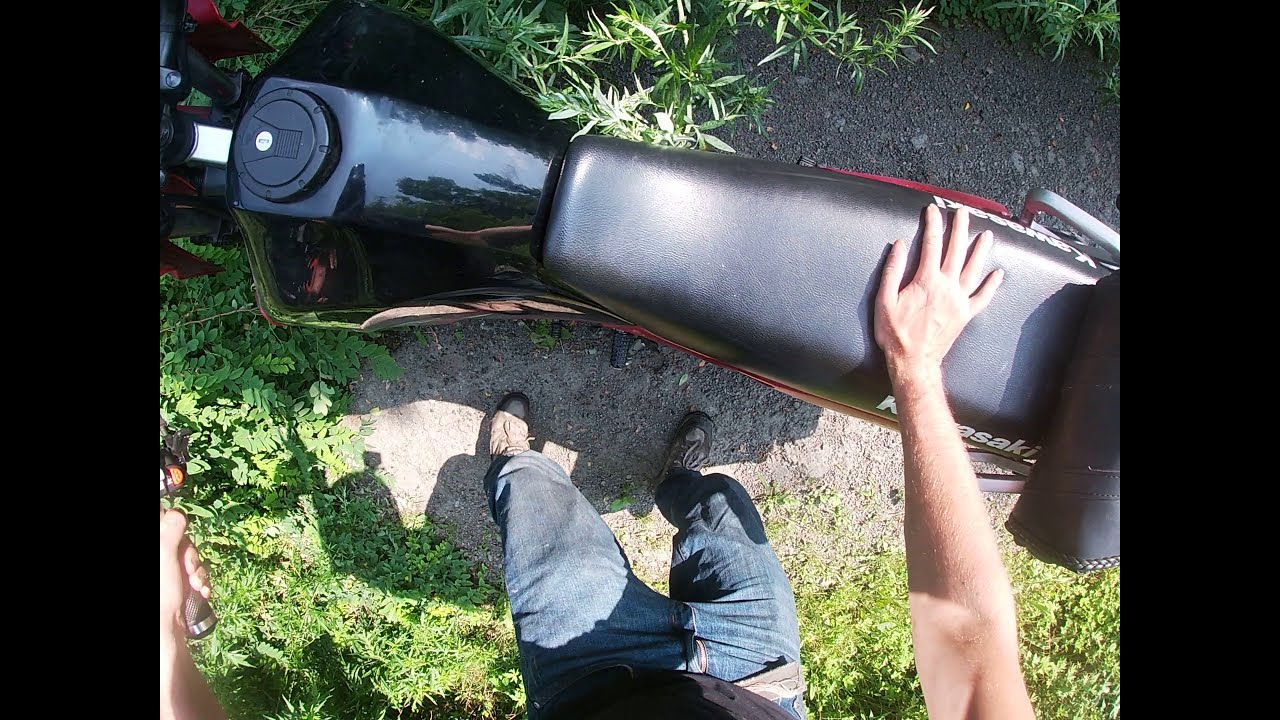In the image, a man stands in a sunny outdoor setting on a dirt path surrounded by green foliage and tiny stones. The perspective of the photograph is from above, revealing the top of a shiny, black motorcycle with a black leather seat. The man, dressed in blue jeans, a brown or black shirt, and gray or faded black hiking shoes, uses his bare right arm to touch the motorcycle’s seat. The left hand, partially visible, appears to hold one of the motorcycle's handlebars. The motorcycle's shadow is clearly cast on the ground, accentuating the bright, sunny day.